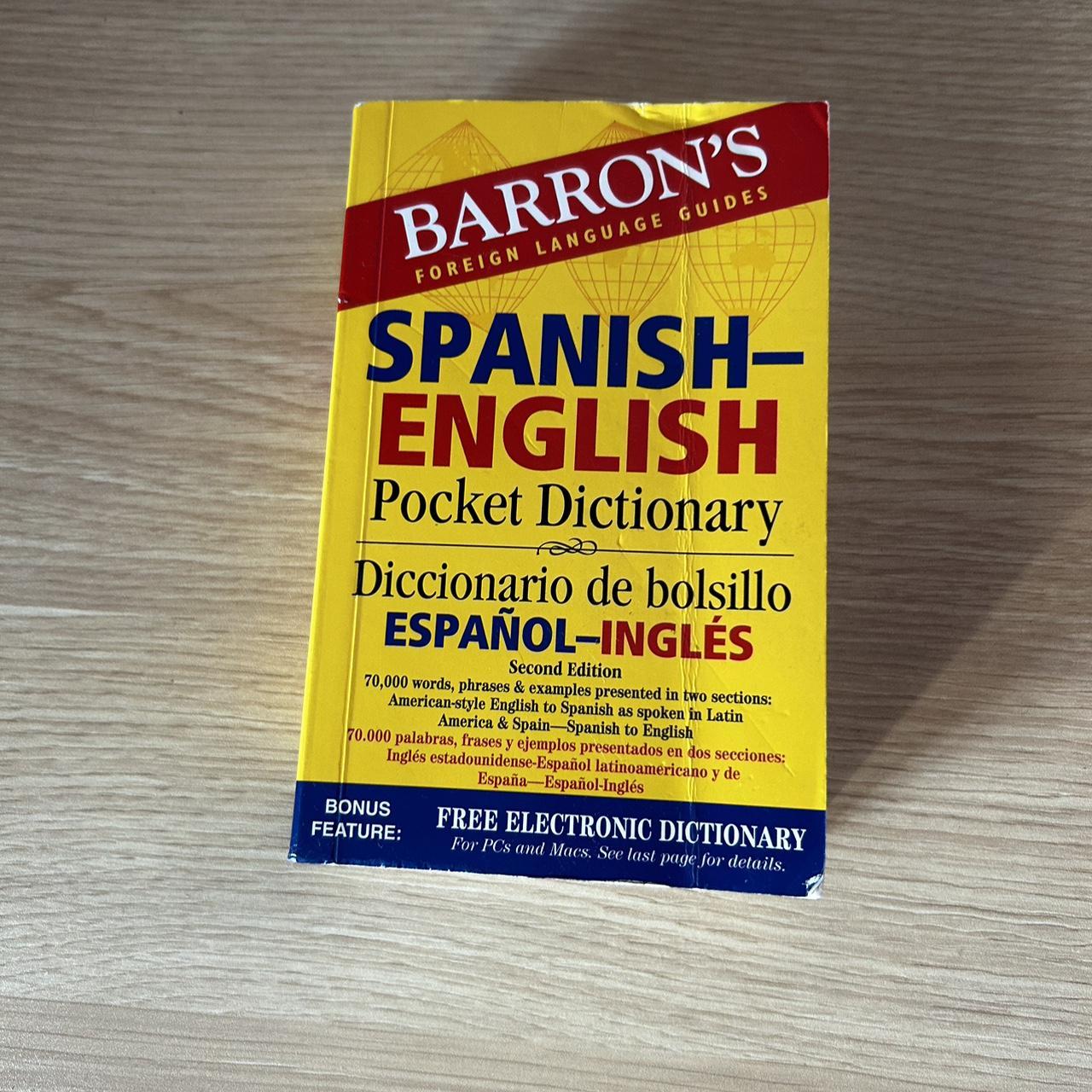The image displays a wooden desk or table with a gray wood grain finish. Lying on the surface is a Barron's Foreign Language Guide Spanish-English Pocket Dictionary. The book cover prominently features the title, "Barron's Foreign Language Guide," printed in white letters on a red strip. Below the title, the word "Spanish" appears in blue text and "English" in red. Additionally, the cover states, "Second Edition: 76,000 Words, Phrases, and Examples Presented in Sections: American Style English to Spanish as Spoken in Latin America and Spain, Spanish to English," both in English and Spanish. At the bottom of the cover, a blue strip highlights a bonus feature, reading, "Free Electronic Dictionary for PCs and Macs, See Last Page for Details." The book itself is primarily yellow, adding a bright contrast to the gray wooden desk.